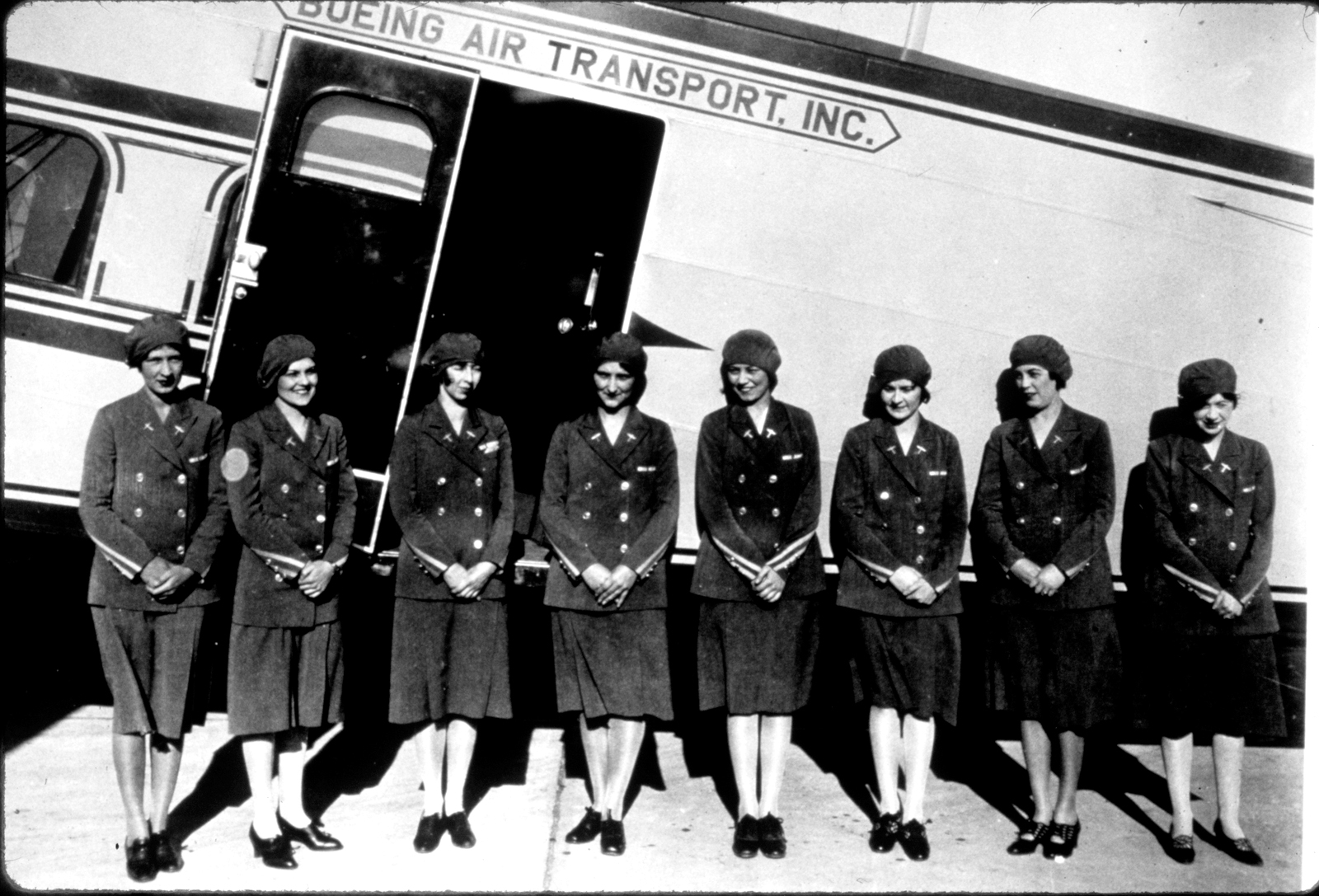This is a detailed black-and-white photograph, likely taken in the 1940s or 1950s. It features eight women, who appear to be flight attendants, all dressed in matching uniforms that include dark skirts falling just below the knees, long-sleeved jackets adorned with double-breasted buttons and stripes on the sleeves, and beret-style caps. Each woman has her hands clasped in front and most are smiling, though their gazes vary, with some looking directly at the camera and others glancing off to the side. They are posing in front of an airplane's fuselage, which prominently displays the inscription "Boeing Air Transport Incorporated." The aircraft, likely white or light-colored, has an open door with a small window, as well as another visible window to the left.